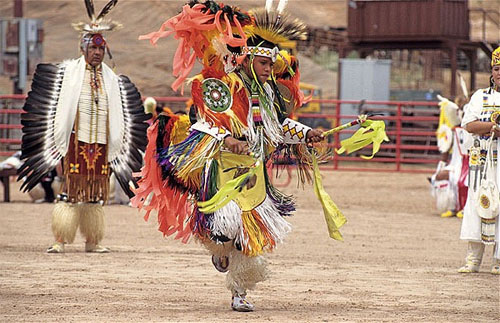The image captures a vibrant scene at a powwow, showcasing the rich culture of Native American tradition. At the center, a dancer dressed in an elaborate multicolored costume adorned with an abundance of tassels, frills, ribbons, and feathers is captured mid-step with his right knee raised and arms outstretched, holding sticks decorated with fabric. His dynamic costume features an official headdress brimming with feathers, exuding an air of ceremonial grandeur.

In the background, to the left, a man stands observing the dance. He is attired in traditional regalia, with wings attached to his arms, a feathered headdress, a coat also detailed with feathers, fuzzy leggings, and traditional shorts. On the right side, a woman in a white leather fringe costume with white boots also observes the scene. The setting appears to be a large dirt field enclosed by cattle gates, further emphasizing the outdoor, communal nature of the powwow.